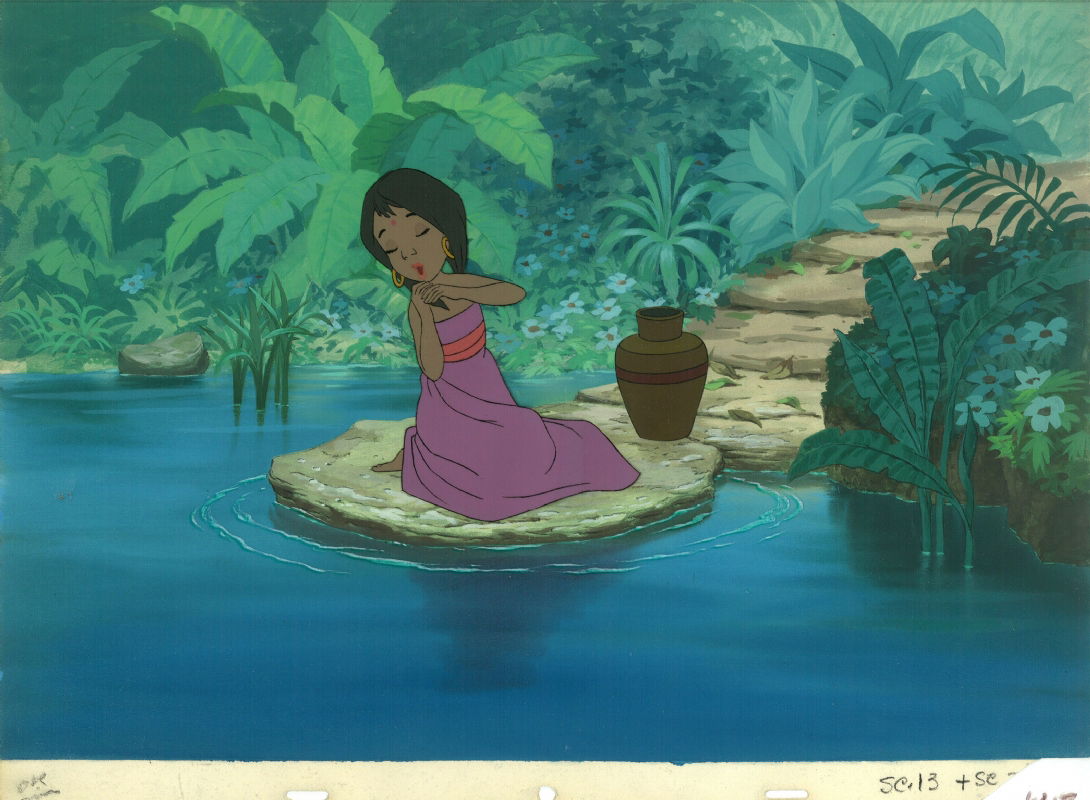In this vibrant and enchanting still from an animated movie, the scene immerses the viewer in a world dominated by soothing blues and lush greens. From the right side of the image, a series of tan oblong steps descend gracefully into a tranquil expanse of smooth blue water, culminating in a larger round step that rests serenely at the water's edge. The presence of minute, delicate ripples around this final step suggests gentle movement within the water, adding a touch of dynamic realism.

The background is a verdant tapestry of blue-green foliage, with an array of plants and trees filling the scene with life and depth. On the last, largest step sits a solitary brown jug, a humble companion to the young girl beside it. She dons a striking purple sleeveless gown cinched with a vivid red sash, her attire contrasting beautifully with her dark skin. Adorning her ears are elegant hoop earrings, and her long braid cascades past her shoulders, framing her serene face.

The girl's pose is one of contemplative grace; her arms are bent, hands tenderly cradling her chin. Her eyes are closed, and her lips part as if caught in a moment of song, evoking a scene of calm and introspective melody. This detailed composition captures both the tranquility of the setting and the emotive depth of the character within it.